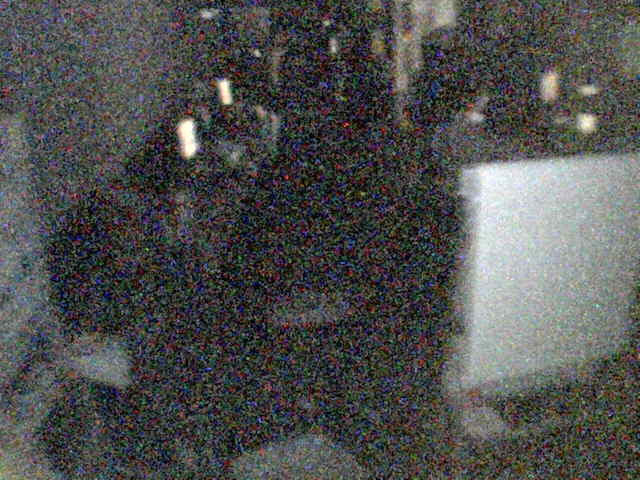The image presented is a heavily blurred and static-filled scene with an indeterminate background. Dominated by a staticky texture, the image features a mix of blue, green, yellow, and black dots that obscure detail. On the right-hand side, a vertically oriented gray square stands out prominently. A similarly gray object is positioned at the bottom, while another gray element, potentially a dresser, is partially visible along the left edge. Towards the top, distant and scattered white orbs of light can be discerned on both the left and right sides. The overall effect is one of indistinct shapes and colors, engulfed in a pervasive static overlay.